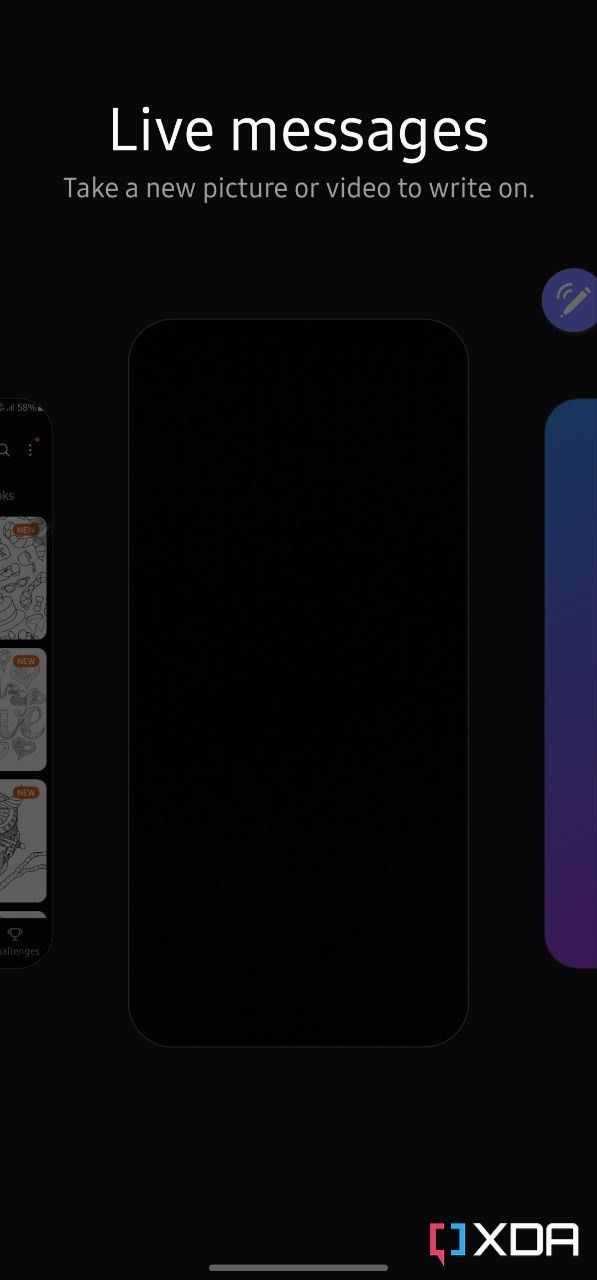This is a detailed description of the image:

The image is a screenshot from the XDA Developers website. In the bottom right corner, the XDA logo is prominently displayed. This logo features two open and close brackets, the first in pink and the second in blue, followed by the text "XDA" in uppercase white letters. At the top of the page, the white text "Live messages" is clearly visible, with a smaller grey subtext beneath that reads "Take a new picture or video to write on." The color scheme of the webpage is predominantly black, giving it a sleek, modern appearance. On the far right edge, there is a faint blue pen icon and a small blue stripe, both of which appear to be slightly greyed out. The overall contents of the webpage are obscured by a black filter, making them not easily visible. The most visible and distinctive element in the screenshot is the XDA logo located in the bottom right corner.